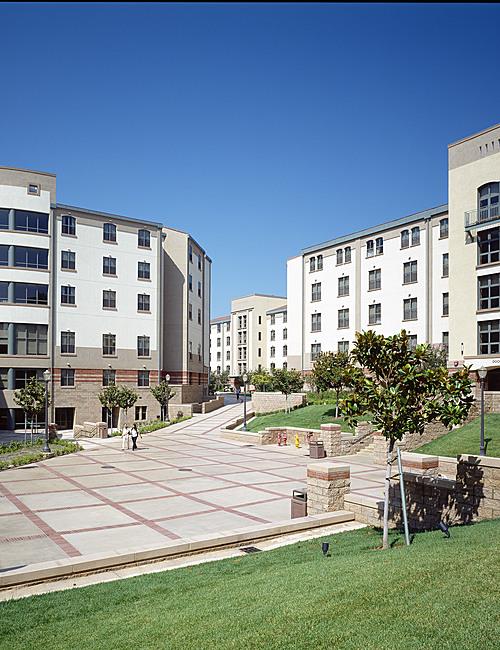In the foreground of this photograph, a mixed patch of green grass, interspersed with lighter and darker shades, and specks of yellowed grass, sets the scene. The background features a line of slender, lush green trees. Nestled amongst the greenery are stone structures, showcasing a textured off-white, tanny color with subtle orange-toned accents. Nearby, a few tan and gray trash cans are positioned next to these stone structures.

The ground below is a stone walkway, meticulously patterned in a brick inlay style. Beyond the walkway rise several large buildings, characterized by an off-white and gray palette with additional sections of brick inlay. One of the buildings, standing out with its sharp lines and stone finish, displays numerous windows. The sky above is a clear blue, casting a serene backdrop to the scene. Below, a handful of people are captured in motion, walking through this well-composed urban landscape.